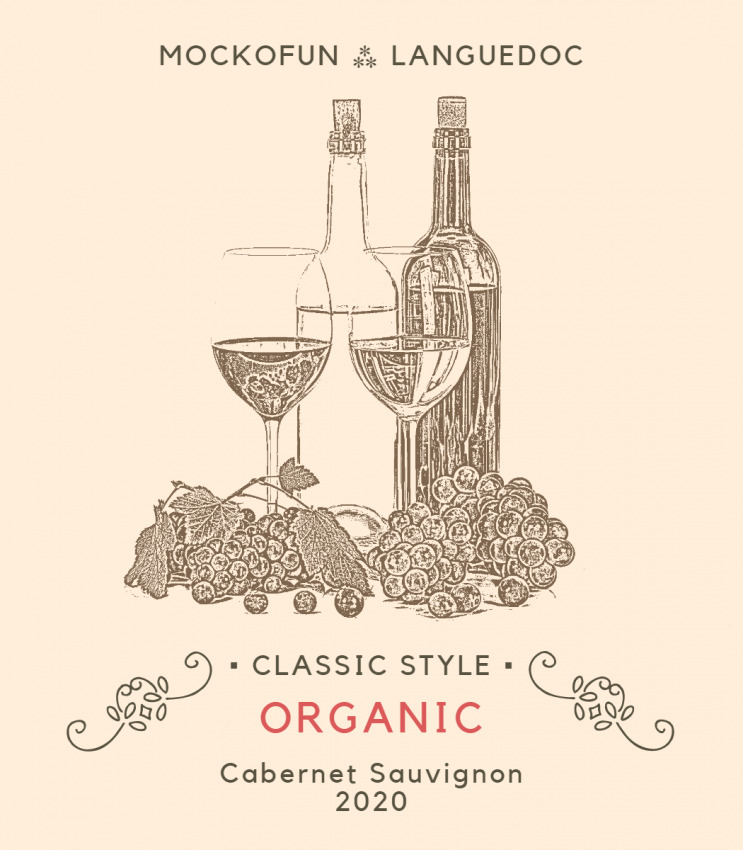The poster for the wine advertisement showcases a sophisticated and elegant design primarily using red and black fonts on a light pink background. Central to the layout is a gray wine bottle flanked by white wine bottles and glasses. At the top of the poster, it reads "Mako Fun Languedoc," and at the bottom, in classic style typography, it states "classic style" and "organic" in red, followed by "Cabernet Sauvignon 2020."

The poster features detailed illustrations of vineyard imagery, including brown images of grapes with grape leaves, and reflections of these grapes are visible in the wine glasses below. There are two prominent wine bottles, one containing red wine and the other white wine, each sealed with corks. This advertisement also includes two wine glasses, each filled with a different type of wine. Flanking the "classic style" and "organic" text are decorative swirl designs, adding an elegant touch to the simplistic yet refined advertisement.